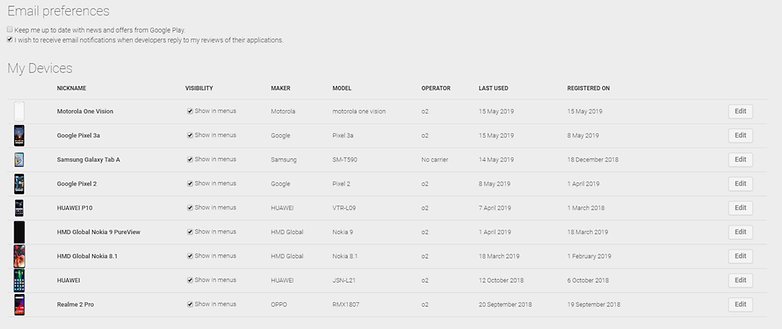This webpage allows users to set their email preferences for various devices. The layout features several columns under the "My Devices" section, each representing different details about the devices. From left to right, the columns include an image representing the device, a nickname for the device, visibility status indicating where the device is shown, the manufacturer, the model name, the operator, the date it was last used, and the date it was registered. The final column on the right side contains an edit button, enabling users to change the device names or nicknames.

The entire page is designed with a light gray background and features black text in a basic font, likely Arial. The first column on the left-hand side displays the images and nicknames of the devices. Each device is listed in a separate row that includes all the aforementioned details, allowing users a clear and organized view of their devices.

At the top of the page, there are two options that users can check or uncheck to customize their email preferences. The first box is labeled "Keep me up to date with news and offers from Google Play." The second box, which is checked in this case, says "I wish to receive email notifications after developers reply to my reviews of their applications."